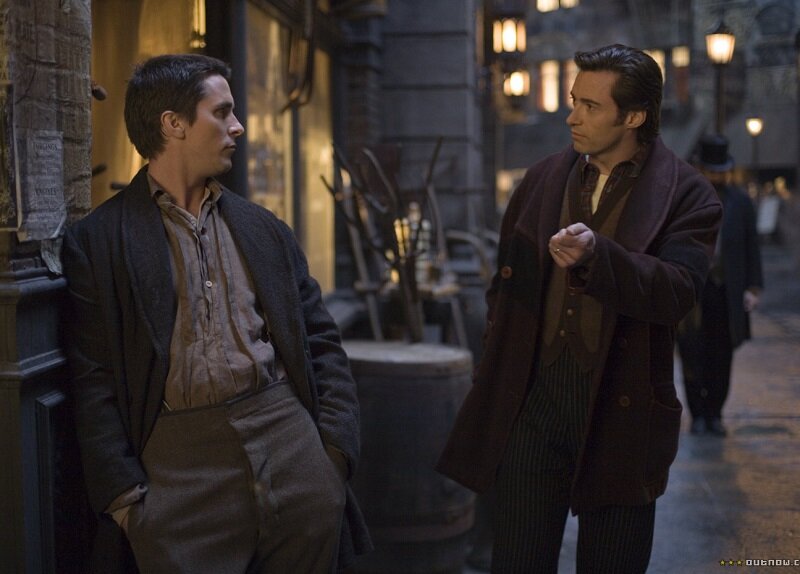This detailed photograph captures a street scene set in what appears to be the late 19th or early 20th century, likely in Europe or the United States, with a strong influence of old England. In the foreground, two men, who bear a striking resemblance to actors Christian Bale and Hugh Jackman, stand engaged in conversation. The man on the left, resembling Christian Bale, has short hair and is dressed in a dark gray coat over a light gray shirt, paired with matching gray pants. He leans casually against a gray brick or wooden building, hands in his pockets, with a wooden barrel behind him. Opposite him, the man resembling Hugh Jackman has short brushed-back darker hair and is gesturing with his left hand. He is wearing a dark jacket, possibly gray or maroon, over a brown vest and black striped pants. The cobblestone sidewalk and blurred streetscape, with elements such as street lamps and multiple buildings with windows, help set the historical ambiance. A third man, situated in the background, wears a tall top hat and full black suit, reinforcing the period setting. The overall scene evokes a cinematic quality, suggestive of a film shoot involving these distinguished actors.